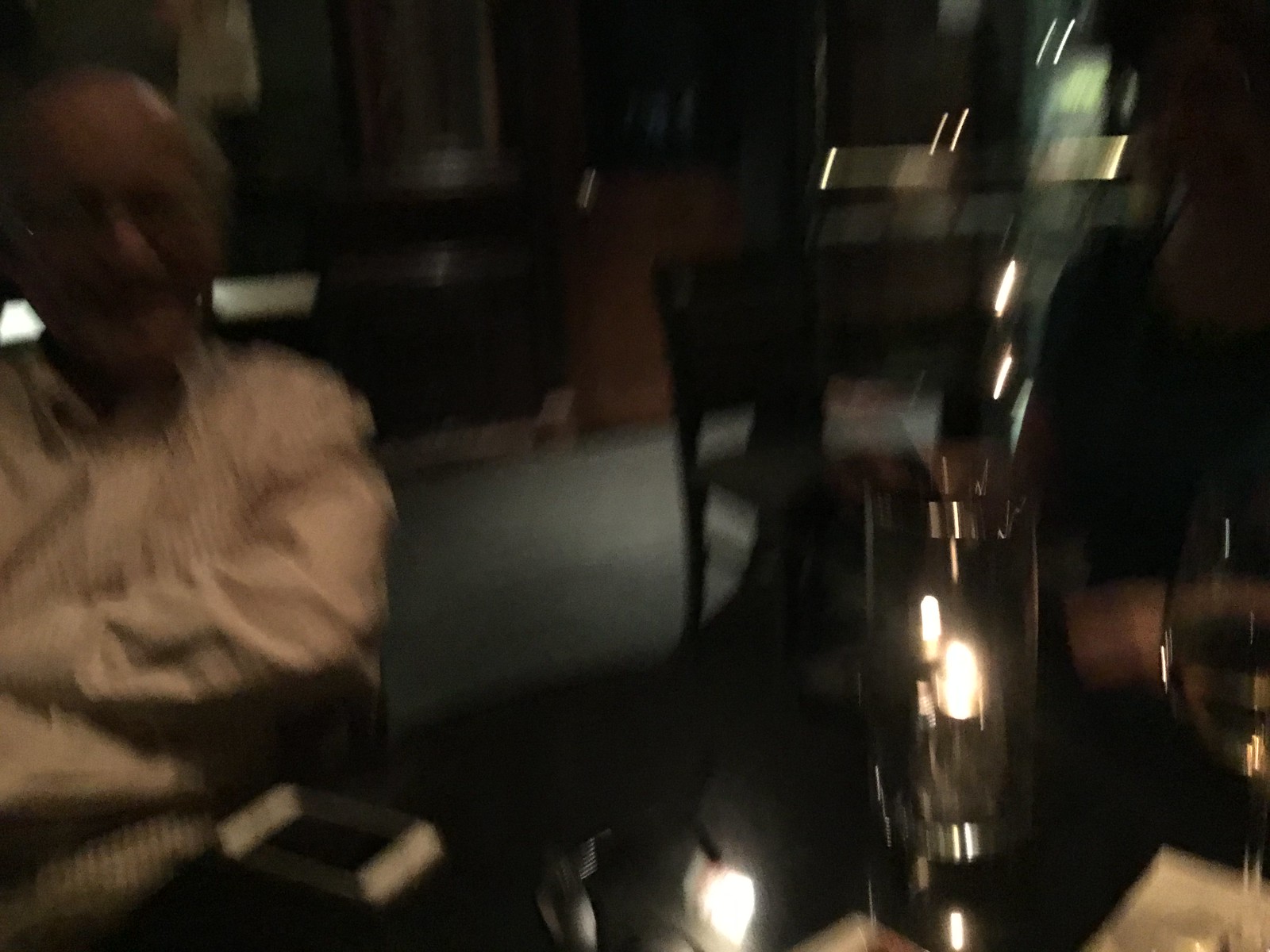The image depicts a dimly lit, out-of-focus indoor scene that could either be a restaurant or a home setting, adding to the ambiguity. Dominating the bottom and right parts of the frame is a dark table. Towards the left, an elderly man, possibly in his 70s or 80s, is seated facing the camera. He’s wearing a light-colored, long-sleeved button-down shirt, which appears to include some checkered patterns. His arms are crossed over his chest, and he sports a bald head with a fringe of gray hair, a beard, glasses, and potentially a mustache, though this is unclear due to the blur. It’s hard to tell if he is smiling or laughing. In front of him on the table lies a white rectangle, likely an older style iPhone. The center of the table is adorned with a tall glass candle holder, resembling a lantern, featuring a chrome-colored metal band at the top and bottom, emanating dim light that reflects off the table surface. Additionally, there's some other source of bright light, possibly another candle, glowing on the table. In the lower right corner, a half-filled stemmed wine glass sits on a napkin, containing what seems to be water or white wine. The background, though indistinct, reveals a second table and a gray carpet, along with either furniture or restaurant supplies, shrouded in darkness and further contributing to the photo's ambiguous atmosphere.